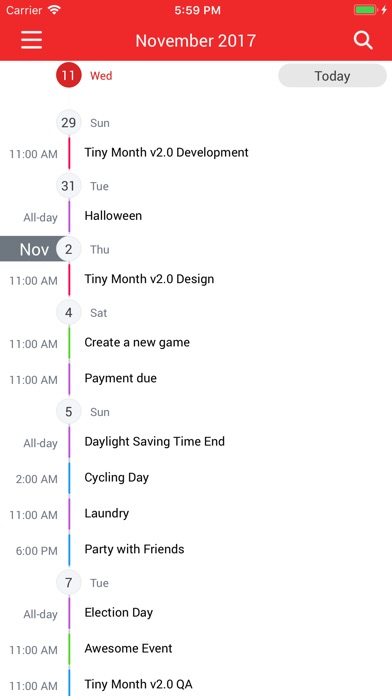This is a detailed screenshot of a mobile phone's display. At the topmost section, the status bar features the name of the carrier inside a red rectangle with white font. To its right, a full Wi-Fi icon indicates a strong network signal. Centrally positioned, the time reads 5:59 PM. Toward the far right, a battery icon filled with green shows it is charging, marked by a white thunderbolt symbol.

Below the status bar, the date "November 2017" is displayed alongside a white magnifying glass icon. The main section of the screenshot is a timeline view of a digital planner or calendar. At the top, in red text, "11 Wednesday" is highlighted, and a small gray oval with darker gray font says "Today."

The timeline commences with "29 Sunday" in black text inside a gray circle, and the day "Sunday" in gray font. Below this entry at 11 AM, there's an event titled "tiny month version 2.0 development." Following this, "31 Tuesday" is listed with an all-day event "Halloween."

Continuing the timeline, "November 2nd Thursday" is mentioned next with an event at 11 AM: "tiny month version 2.0 design." Subsequent to this is "4 Saturday," featuring two events at 11 AM: "create a new game" and "payment due."